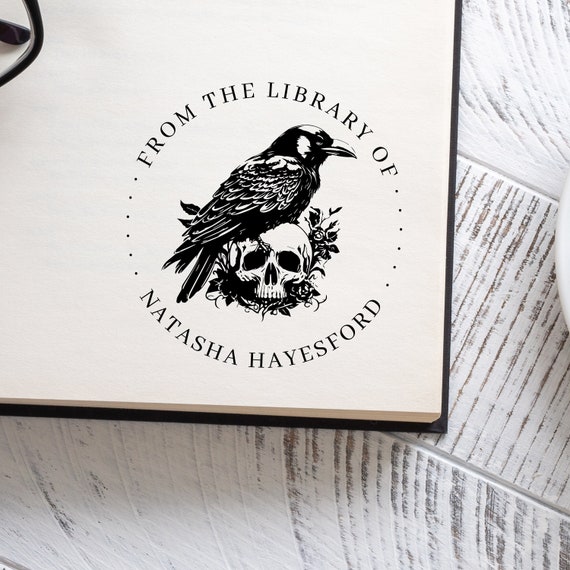In the image, a book with a black binding and possibly a black string bookmark is open, displaying its cream-colored first page on a white wooden slat table. Prominently featured on this page is a black and white sketch of a raven with distinctly pronounced feathers, sitting on a skull. The raven, facing east with a long beak and black eyes, grips the top of the skull with its foot. Surrounding the skull are some small roses and possibly some dried reeds. Encircling this macabre illustration is the text, "From the Library of Natasha Haysford" within a circular stamp. Additionally, a pair of black-framed glasses can be seen at the upper left-hand corner of the page.